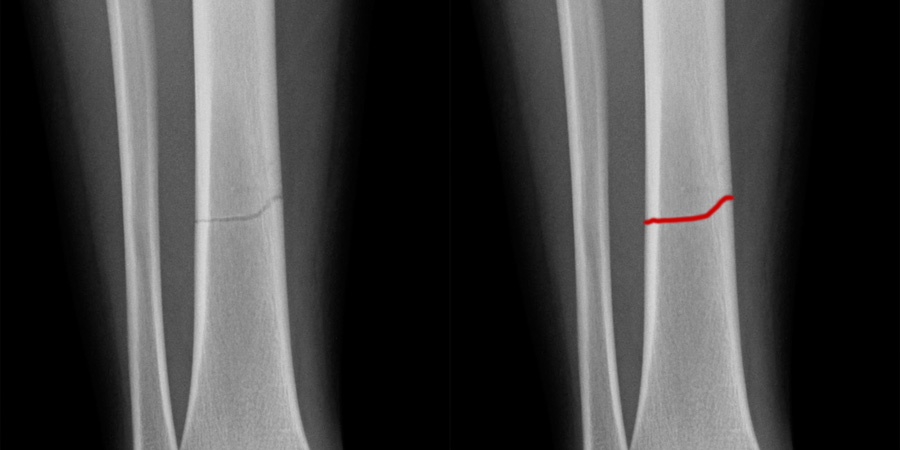The image consists of two x-ray scans of what appears to be a lower leg, specifically focusing on the tibia and fibula bones. Both x-rays are set against a completely black background, enhancing the contrast of the skeletal details. The x-ray on the left shows a clear view of the bones, with the larger tibia on the right side and the smaller fibula on the left. A distinct dark gray line, indicating a fracture, runs horizontally through the center of the tibia. The x-ray on the right is an identical scan, but the fracture is emphasized with a red line highlighting the crack, making it unmistakably clear. The muscles surrounding the bones are visible as darker gray areas. These detailed images unmistakably show the fracture, making it apparent even to the untrained eye.